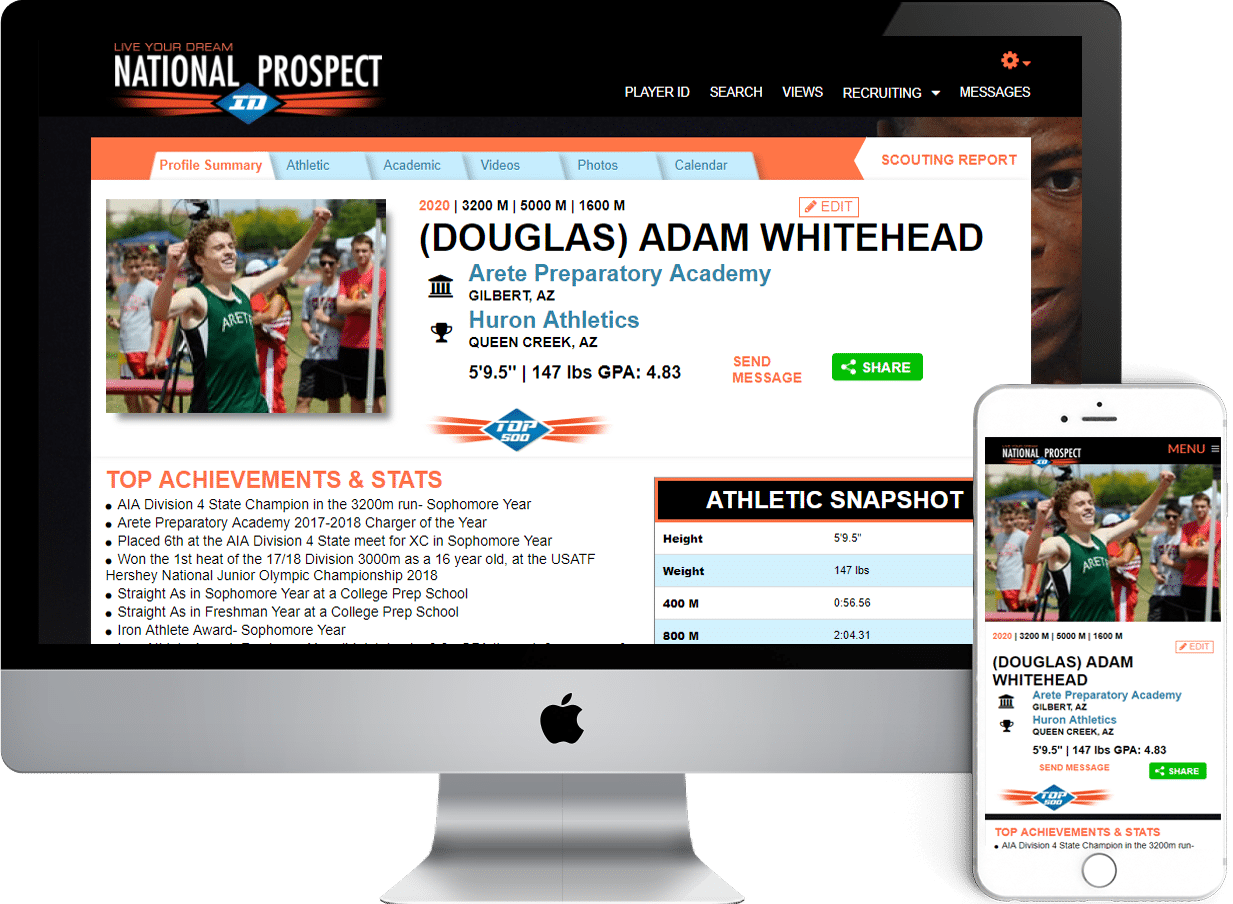A meticulously designed flat-screen monitor dominates the image, featuring a sleek, white, metal finish. Prominently branded with Apple's logo at the bottom, it stands on a minimalist 'foot.' The monitor's realistic appearance hints at computer-generated perfection. Adjacent to its bottom right corner is a cell phone.

The monitor's screen displays a fitness-oriented dashboard from 'National Prospect ID' under the tagline "Live Your Dream," located in the upper left corner. In the upper right corner, the interface includes 'Player ID,' 'Search Views,' and 'Recruiting' options, alongside a 'Messages' section. A settings icon in orange features a downward menu.

The central dashboard highlight includes tabs: 'Profile Summary,' 'Athletic,' 'Academic,' 'Videos,' 'Photos,' and 'Calendar.' The 'Scouting Report' tab sits isolated at the far right. The 'Profile Summary' tab is active, marked by its white background and orange font, while the rest remain blue.

In this active section, a photograph of a youthful male athlete is prominently displayed. He sports a green tank top with partially visible white text, possibly "ARET." His appearance is marked by a fair complexion and reddish-brown hair. Accompanying the photo are details about his athletic achievements: "2020, 3200M, 5000M, 1600M." The athlete's profile is named 'Douglas Adam Whitehead,' with an 'Edit' button for profile modifications.